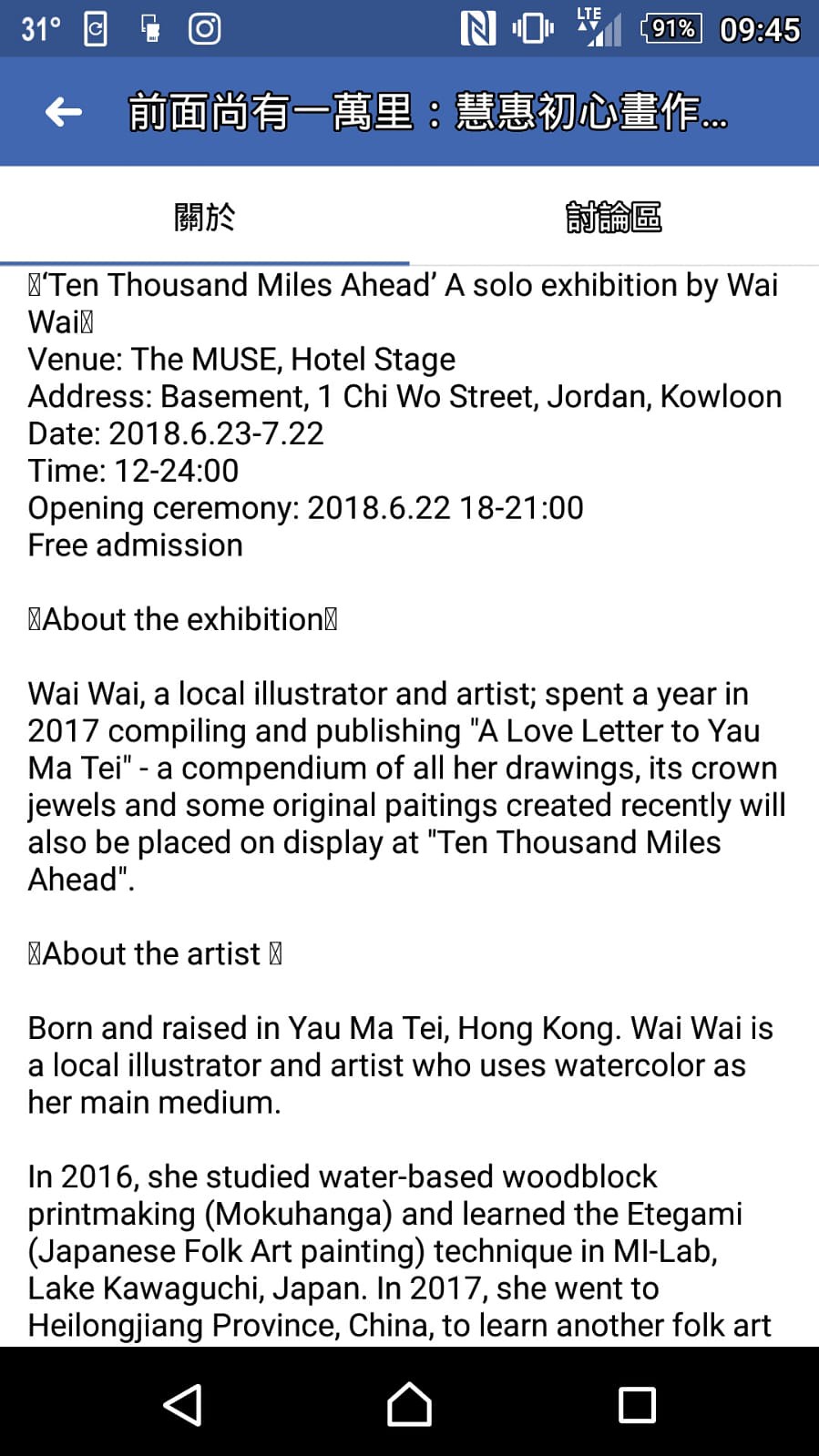This screenshot appears to be from an Android device displaying a promotional flyer for an art exhibition. The top of the screen shows typical smartphone elements, including the time (9:45) on the right, a battery status of 91%, and cell signal strength. The temperature, 31 degrees, is noted in the top left. The screen includes navigational tabs written in Chinese, with the left tab highlighted. Below the tabs, the flyer features both Chinese symbols and English text.

The main event is titled "10,000 Miles Ahead: A Solo Exhibition by Wai Wai." The exhibition will be held at the Muse Hotel Stage, located at Basement 1, Chai Wo Street, Jordan, Kowloon. The exhibition dates are from June 23, 2018, to June 27, 2018, with the opening ceremony on June 22, 2018, at 9:00 PM. Admission is free.

The flyer provides a brief description of the exhibition, stating that Wai Wai, a local illustrator and artist, spent a year in 2007 compiling and publishing a love letter to Yau Ma Tai, a compendium of her drawings. The exhibition will feature these works along with some original paintings created recently.

At the bottom of the screen, a black bar features icons for back, home, and share functions, set against a consistent design of black-and-white graphical elements.